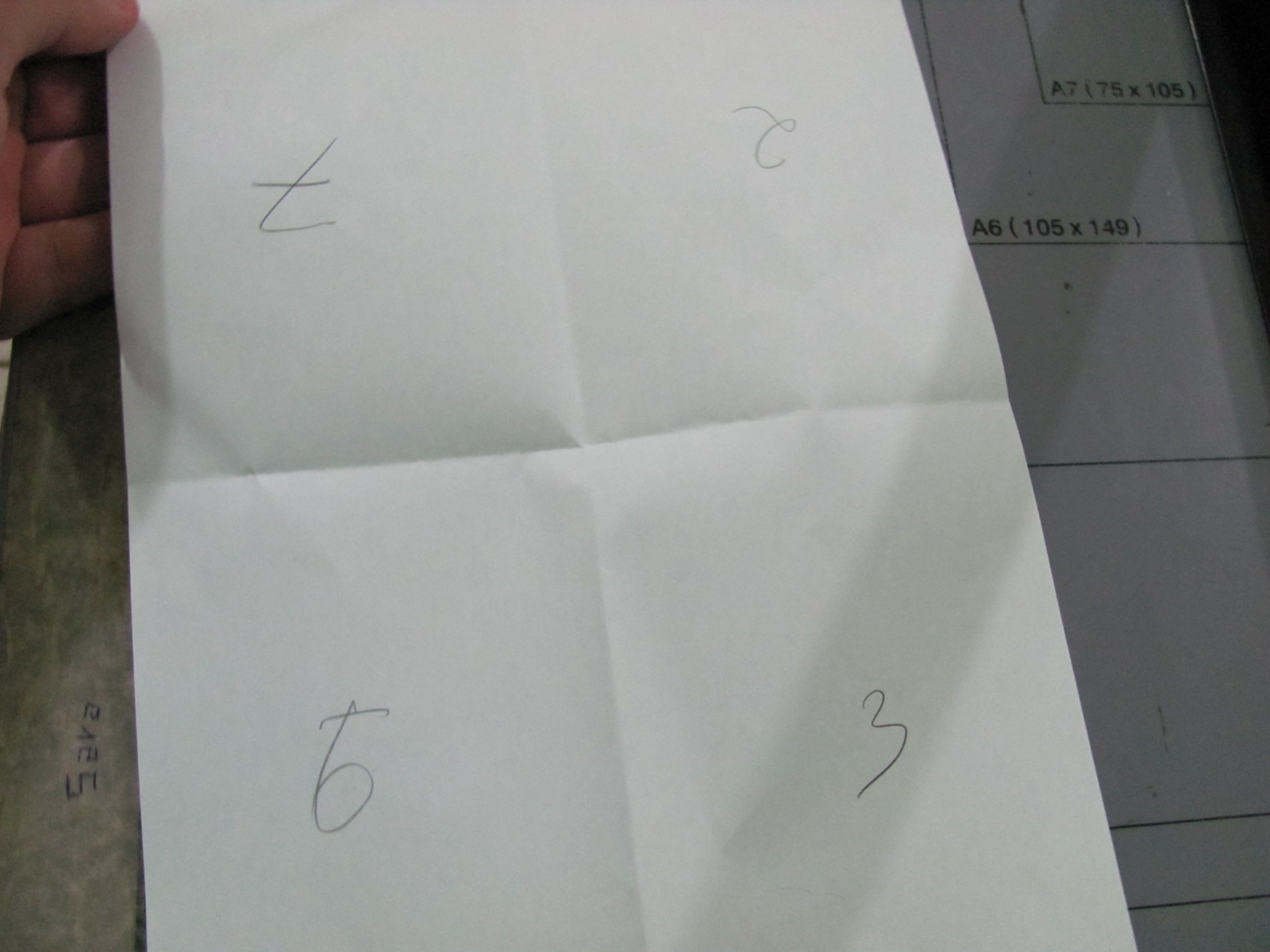A crisp white sheet of standard printer-sized paper, evidently folded into quarters, lies at the center of the image, revealing distinct vertical and horizontal creases that divide it into four equal sections. Handwritten in pencil are the numbers 6 in the bottom left corner, 3 in the bottom right corner, 7 (upside down) in the top left corner, and 2 (upside down) in the top right corner. A person's hand is visible, holding the paper at the top left corner. The hand displays the thumb, middle, ring, and pinky fingers, with the index finger cut off by the top edge of the picture. The thumb slightly overlaps the paper's front while the rest of the fingers are positioned behind it.

In the background, partially obscured by the focal paper, are additional sheets covered with mathematical equations. On the right-hand side, a white paper features various sizes of squares and two prominent equations: "A7 (75 x 105)" and "A6 (105 x 149)." To the left in the background, another sheet carries a blurred equation, rendering it illegible but suggesting further mathematical context. The overall scene appears to be set in a studious environment, potentially amidst problem-solving or homework activities.